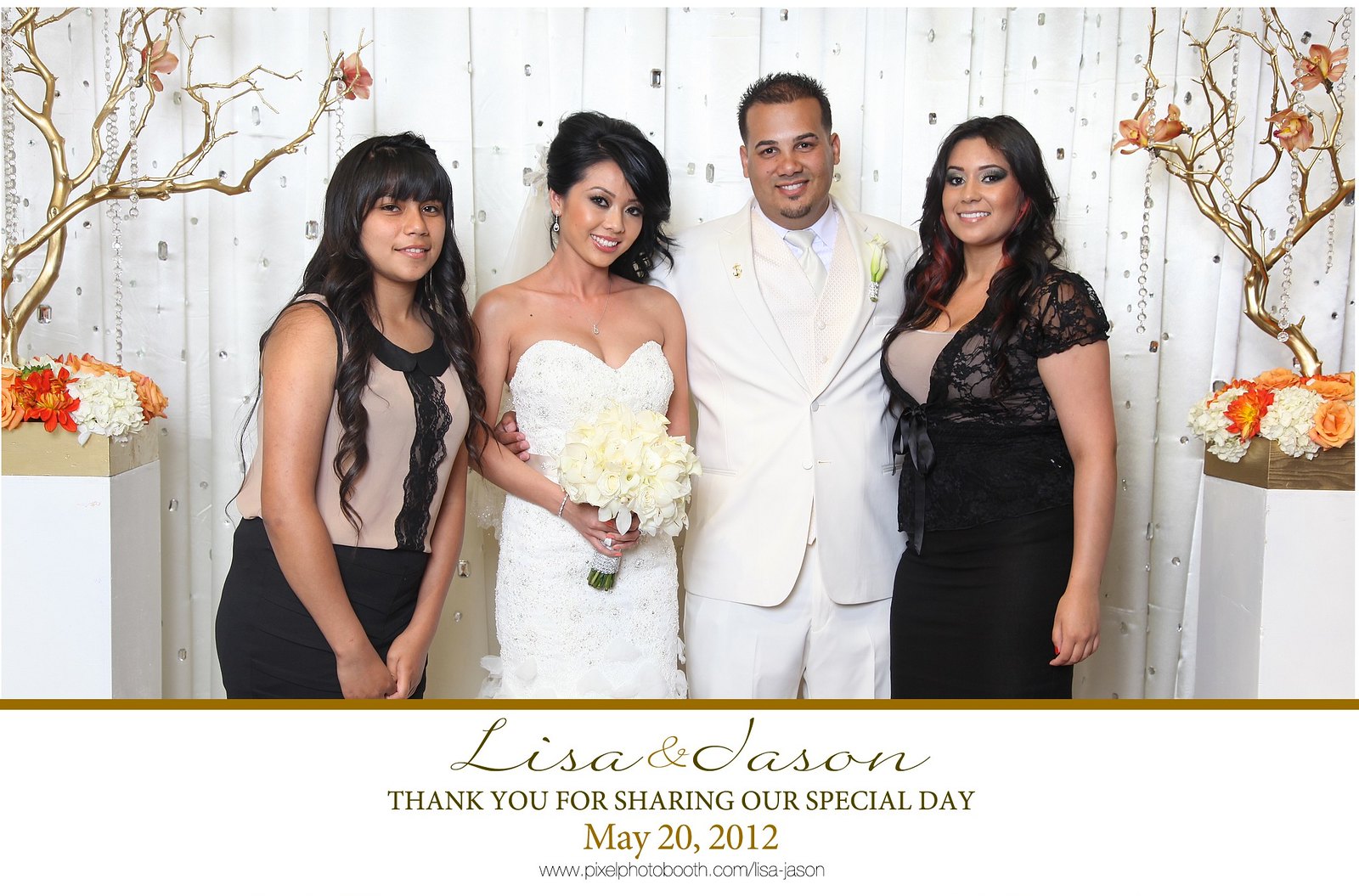This professionally-taken wedding photo captures a beautiful moment shared by four people, arranged against an elegant backdrop of a white jeweled curtain and golden branches adorned with flowers in white vases on either side. Centered in the image are the bride and groom, with the bride dressed in a stunning strapless bejeweled gown and holding a bouquet of white lilies, and the groom donning a white suit with a white tie, complemented by a white corsage. The bride, who appears to be of Asian descent, and the groom, who has a slight beard and appears to be Hispanic, stand smiling at the camera. Flanking them are two women: to the bride's left is a teenage girl with long, dark hair, wearing a sleeveless brown shirt with black lace and a black skirt; to the groom's right is a young woman with long, dark hair, dressed in a black lace top over a beige shirt, also paired with a black skirt. The photo is captioned in the lower center with the text, "Lisa and Jason, Thank you for sharing our special day, May 20, 2012" along with a website link, www.pixelfotobooth.com.